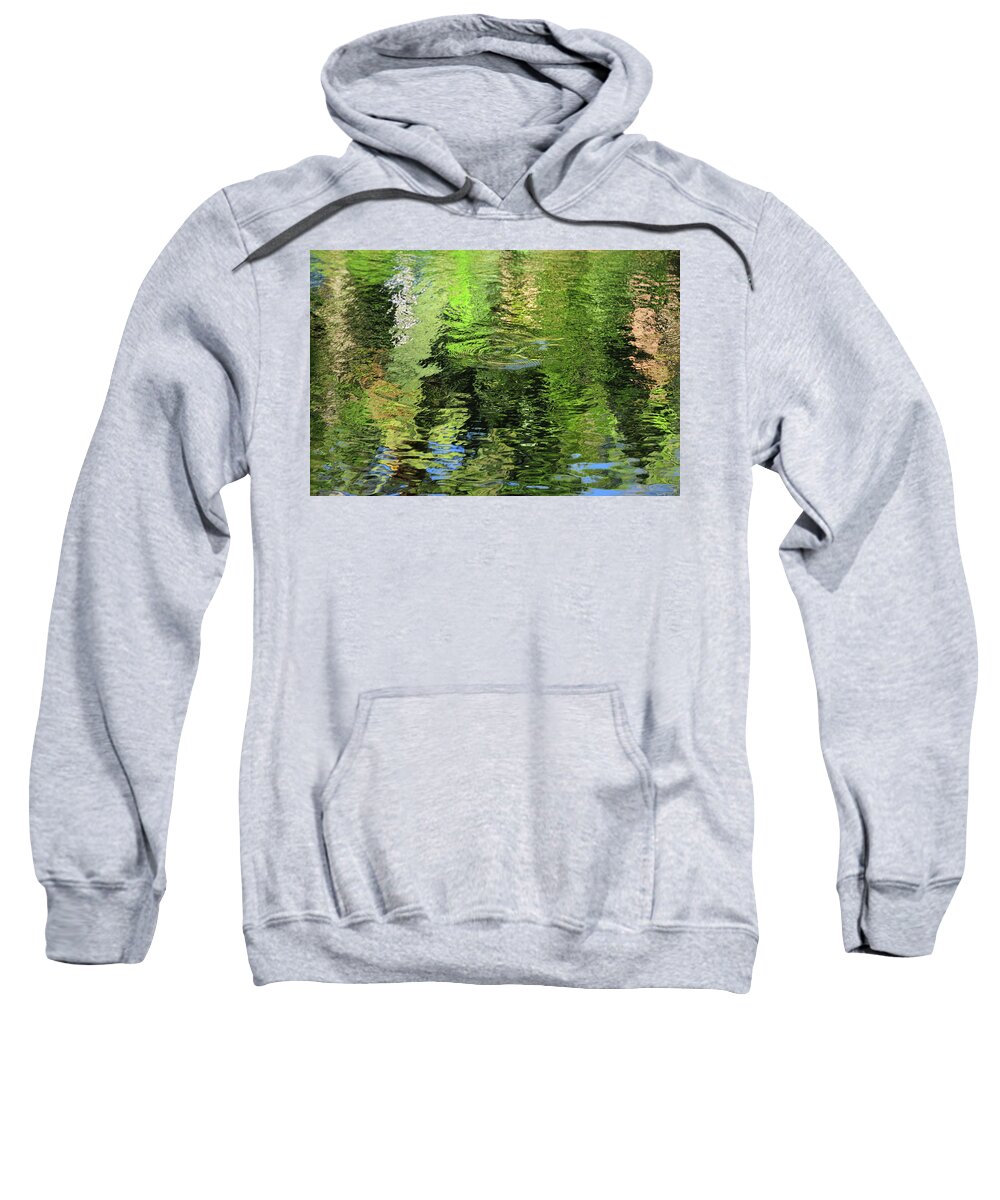The image depicts a digital product advertisement featuring a full-sleeved hoodie jacket. The hoodie, predominantly light green in color with contrasting black drawstrings at the neck, boasts two pockets located at the stomach area for practical hand storage. A notable detail is the square-shaped image emblazoned on the chest, showcasing a serene natural scene: a pond with gentle ripples reflecting lush green trees and a blue sky tinged with sunlight. Also visible are water reeds and blooming plants flanking the pond, adding a touch of flora to the tranquil waterbody. The background of the advertisement is a clean white, ensuring the hoodie and its intricate design stand out vividly.